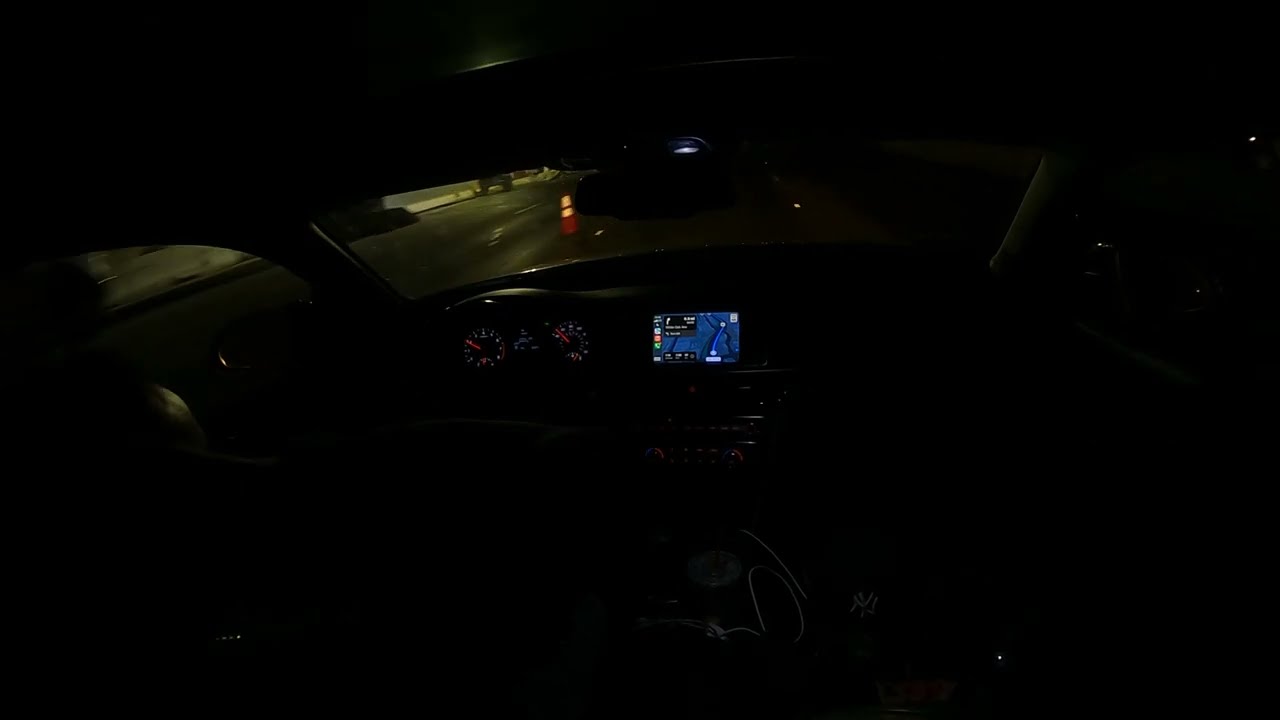The image captures the dimly lit interior of a car driving at night, with most of the scene shrouded in darkness. Despite the low light, several key details are visible. On the left side, where the driver should be seated, the car speedometers and an RPM gauge are illuminated with white numbers, forming two distinct circles. To the right of these gauges, a built-in electronic GPS system is prominently displayed in the middle of the dashboard, casting a bluish hue and showing a detailed map with various shades of blue and small black instruction boxes. Through the windshield, an orange and yellow reflective traffic cone can be seen along with the dark black road the vehicle is traveling on. The far left of the image hints at walls running alongside the road, with no other cars in sight.